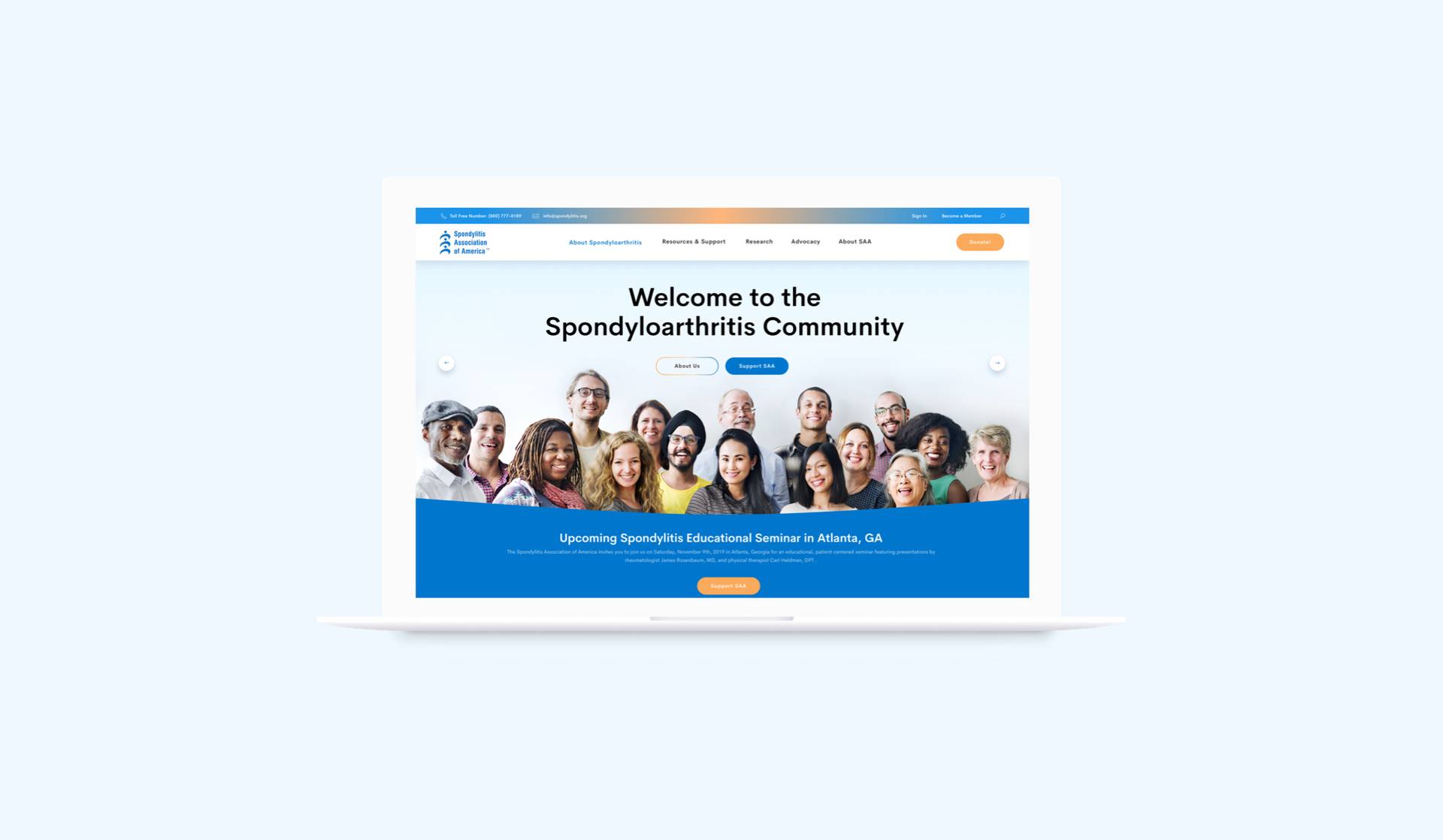On a light blue background, the image prominently features a front view of an open white laptop, displaying the edge of the keyboard and the white bezel. The laptop screen showcases the homepage of a website. At the top of the screen, a blue and orange banner displays a logo. Just below it, a white banner features a blue logo in the corner with the text "Spondyloarthritis Association of America." Black text runs across this banner with an orange button on the right side. Below this, a photograph depicts a group of smiling people seen from the shoulders up, standing before a light blue wall. Above their heads, the text "Welcome to the Spondyloarthritis Community" is written in black. Underneath the photograph, there are two buttons: one outlined in a rainbow color labeled "About Us" and a blue button with unidentifiable white text. Further down, the background turns blue with white text announcing "Upcoming Spondyloarthritis Education Seminar in Atlanta, Georgia." At the bottom center of the screen, an orange button with white text is visible.